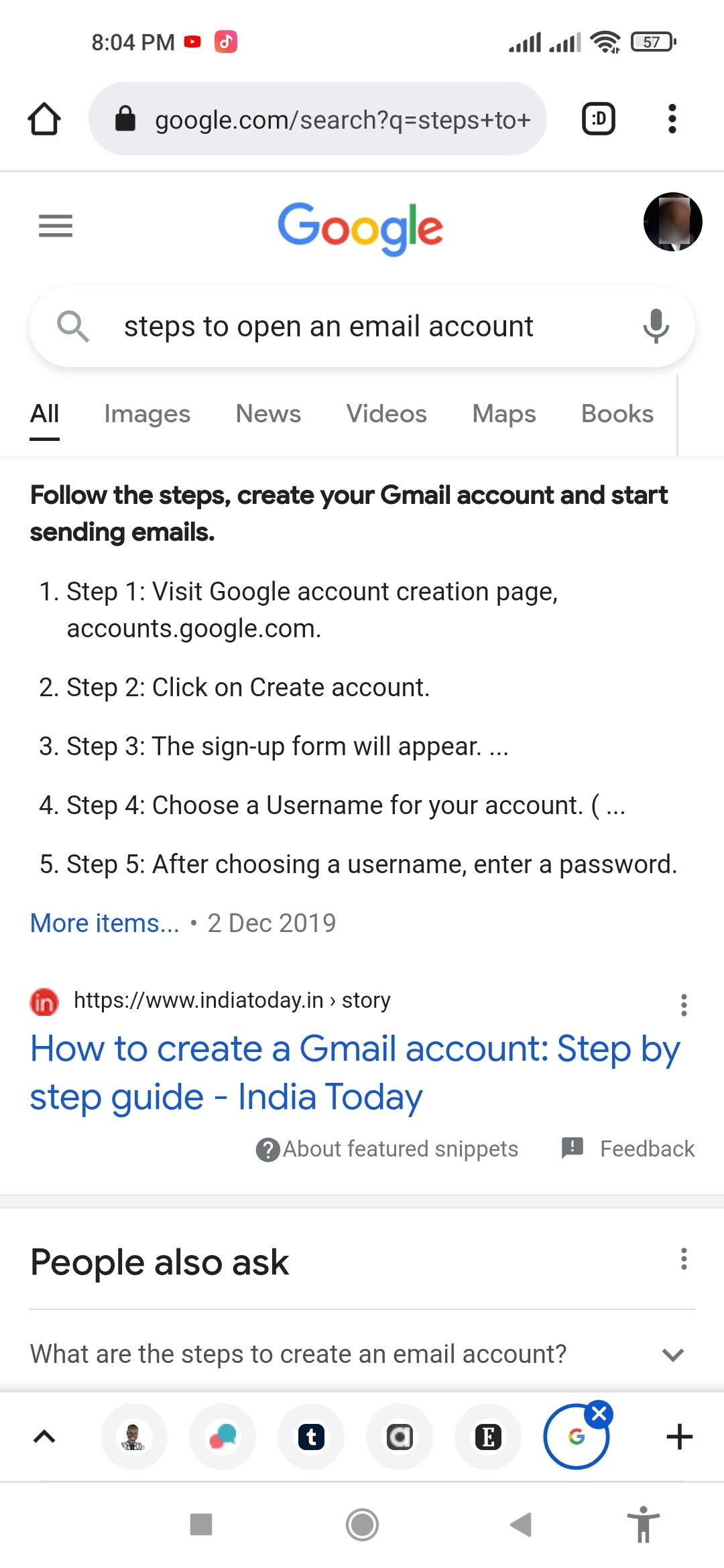The image presents a detailed screenshot of a Google search result on a white background taken at 8:04 PM. The top of the screen shows a small red notification box, followed by a pink notification box containing something white. Below this, there's a small house icon, a Google search button, and a profile icon with a sideways face next to three vertical dots. 

Further down, the screen displays Google's signature logo with three horizontal lines in blue, red, yellow, and green, accompanied by a small circle embedding another image.

The main content of the page features a header reading "Steps to Open an Email Account," encircled in a box that includes tabs labeled "All," "Images," "News," "Videos," "Maps," and "Books." 

Below this header, there is a step-by-step guide on how to create a Gmail account, which includes:

1. Step 1: Visit the Google account creation page at accounts.google.com.
2. Step 2: Click on "Create Account."
3. Step 3: A sign-up form will appear.
4. Step 4: Choose a username for your account.
5. Step 5: After choosing a username, enter a password.

The section ends with a note stating, "More items, 2nd December 2019," followed by a link to an article from "India Today" titled "How to Create a Gmail Account, Step by Step Guide."

At the bottom of the image, common search queries similar to the original one can be seen under "People also ask for the steps to create an email account." Lastly, various navigation icons are aligned at the bottom, including an X mark over the Gmail icon.